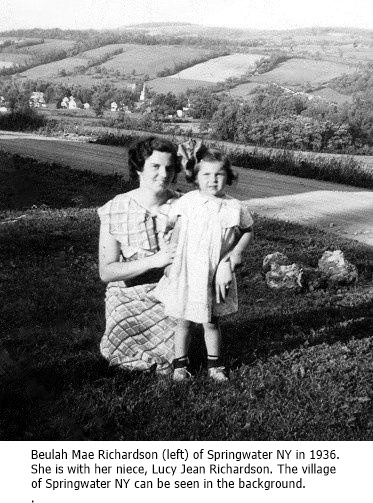This black-and-white photograph from 1936 captures Belula Mae Richardson, kneeling on the grass in a plaid dress with curly dark hair, and smiling as she holds the arm of her young niece, Lucy Jean Richardson. Lucy, who is dressed in a white dress with a ribbon or hat in her short brown hair, stands solemnly at her aunt's side. The scene is set in a grassy field with two visible rocks on the ground, leading to a dirt road. In the background, the hilly terrain of Springwater, New York, can be seen, dotted with farmland, trees, and houses, depicting the rural nature of the village. The caption at the bottom of the photo reads: "Belula Mae Richardson, left of Springwater, New York in 1936. She is with her niece, Lucy Jean Richardson. The village of Springwater, New York can be seen in the background."